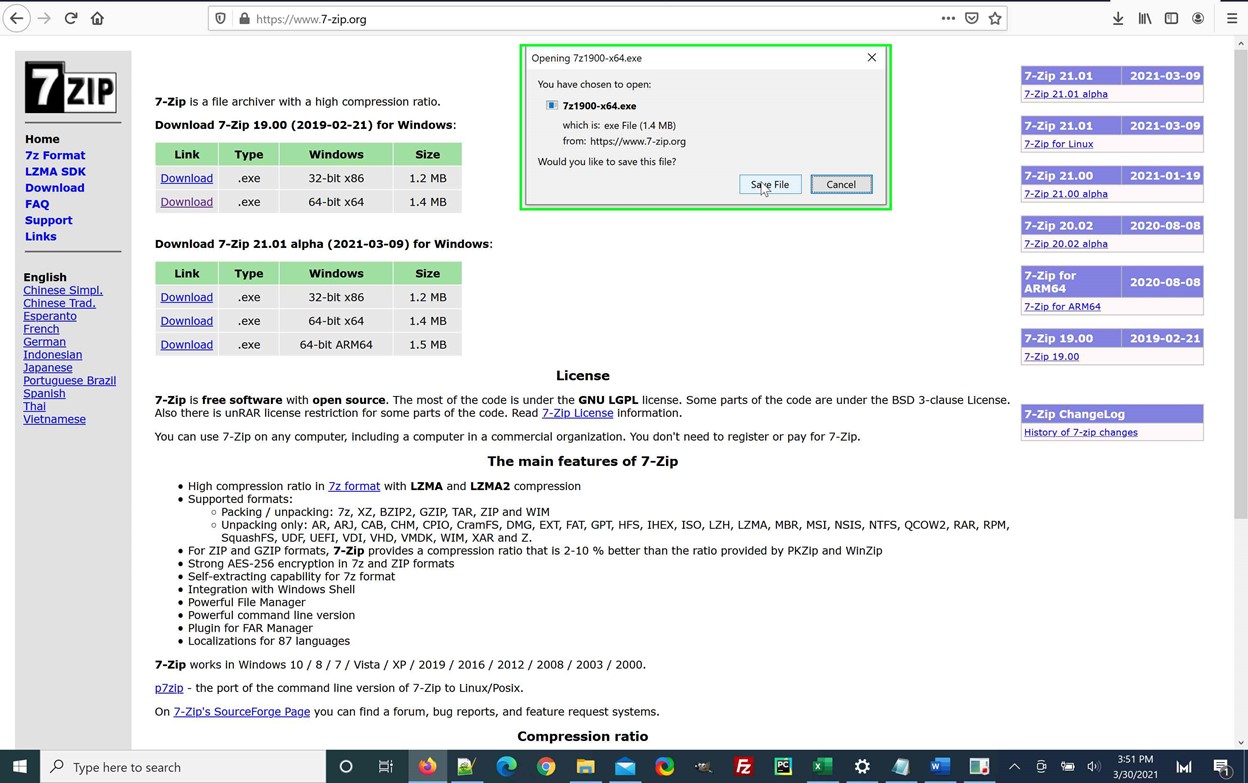The web page for 7-Zip, located at https://www.7-zip.org, features a clean and organized layout designed primarily for users seeking information on the compression software. The left column of the page is shaded in light gray and populated with purplish-blue hyperlink text. This navigation column includes several categories under 'Home' such as 7-Z Format, LZMA, SDK, Download, FAQ, Support, and Links, making it easy for users to find specific information. Below these categories, the page offers a selection of languages for users, with English currently selected. Other available languages include Chinese Simplified, Chinese Traditional, Esperanto (assumed based on partial visibility), French, German, Indonesian, Japanese, Portuguese (Brazil), Spanish, Thai, and Vietnamese, catering to a diverse range of users worldwide.